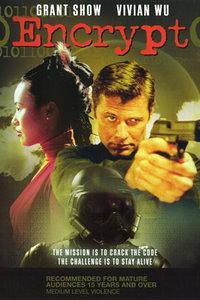This image appears to be the cover of a straight-to-DVD or Blu-ray movie with a distinct low-budget vibe. The background is olive green with a sunburst effect that adds some visual depth. At the top, in white all-caps, are the names of the two leading actors: Grant Show on the left and Vivian Wu on the right. Below their names, the title "ENCRYPT" is prominently displayed in a red thriller-type font, with the final "P" being noticeably bolder.

The central image features a man reminiscent of a James Bond character. He is Caucasian with dark brown hair, wearing a dark greenish or brown long-sleeved shirt. He stands facing the viewer, arms extended, holding a handgun directly aimed forward. His head is slightly tilted down with a serious expression.

To his left and slightly behind him is a profile view of an Asian woman, presumably Vivian Wu. She has black hair styled in a neat, pulled-back fashion, revealing an earring in her left ear. She wears a red top and is looking to the left side of the frame.

Beneath the man and slightly under his right shoulder, there is a mysterious figure clad in black, resembling either a robotic or monstrous entity with a completely covered face, suggesting a mask or helmet, possibly evoking a Stormtrooper comparison.

At the bottom, in small white text, a tagline reads: "The mission is to crack the code. The challenge is to stay alive." This adds an additional layer of intrigue and hints at the film’s thriller elements.